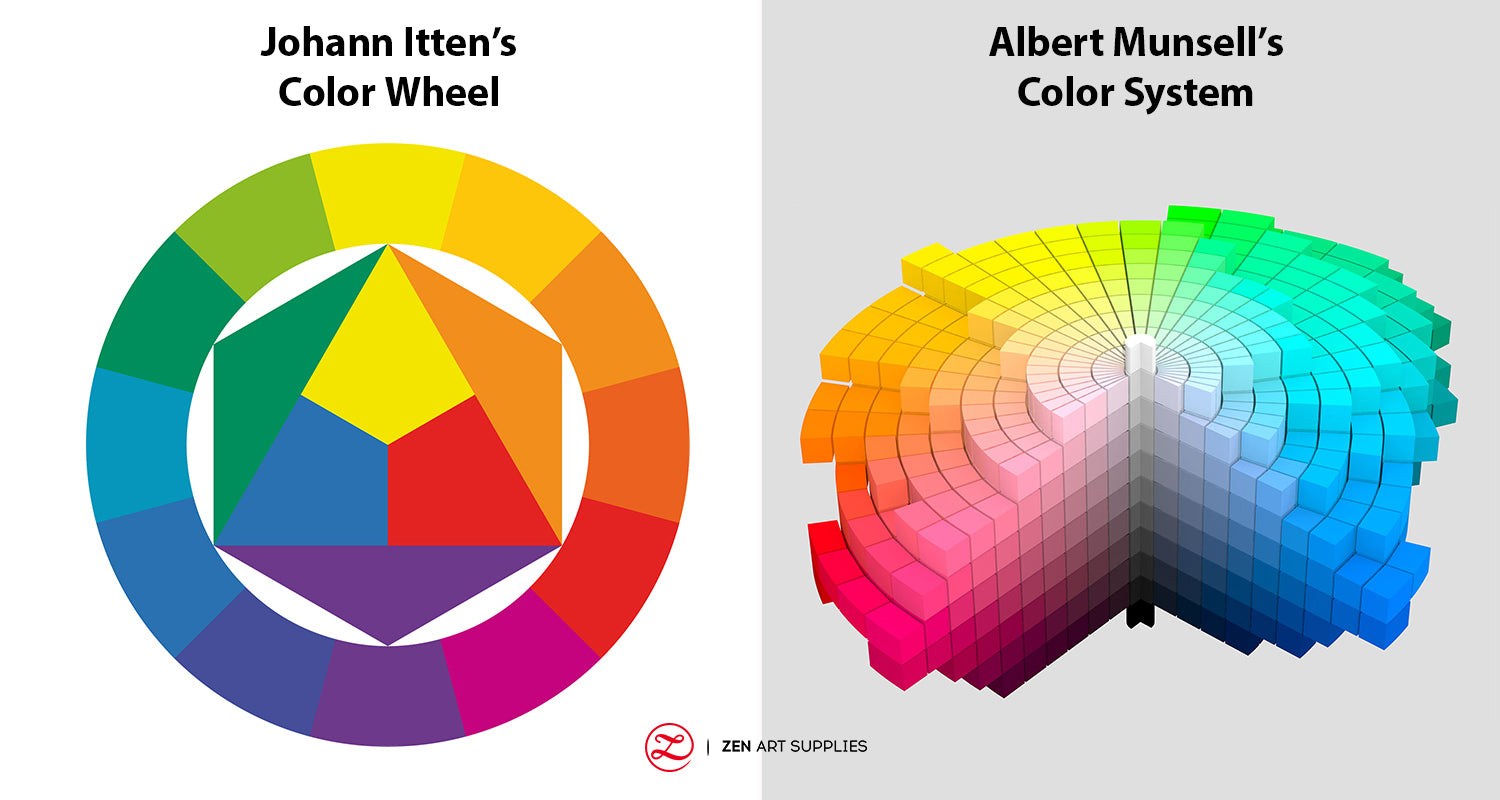This image features two adjacent color wheels, each distinctly labeled and presented in different dimensions. On the left, John Iton's color wheel is two-dimensional, with bold black text at the top center reading "John Iton's color wheel." The wheel starts with yellow at the top and transitions counterclockwise through gold, orange, red, pink, purple, blue, and various shades of green. Within this wheel, the primary colors are arranged in an inner triangle, while the secondary colors form an outer hexagon with their points directed towards the corresponding colors within the wheel. The background of this section is white, providing a clear contrast.

On the right side, Albert Munsell's color system is displayed with a 3D representation in a gray background. The label "Albert Munsell's color system" appears at the top center in black text. This wheel similarly transitions through yellows, greens, blues, purples, pinks, and oranges. The 3D depiction shows varying color saturations, with the colors becoming less saturated towards the center and more saturated towards the edges. This versatile representation highlights the depth and complexity of Munsell's color system, contrasting with the geometric simplicity of Iton's design.